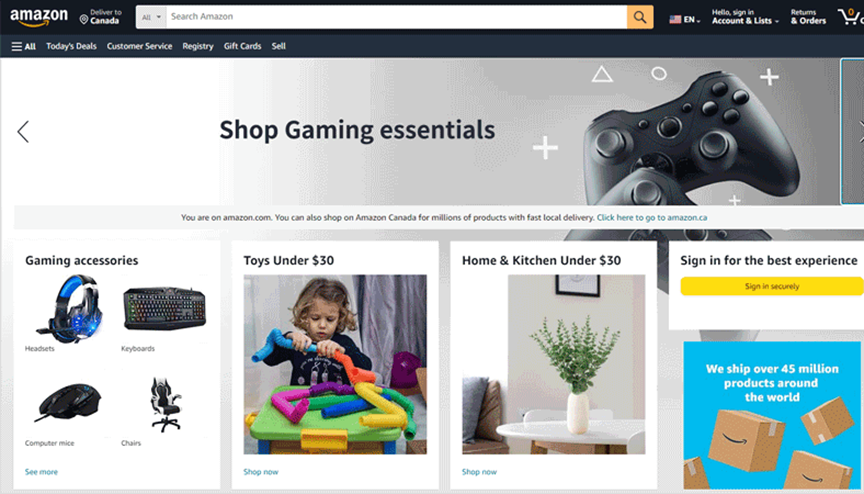The image displays a shopping site on Amazon with a detailed layout. At the top, there's a black banner featuring the Amazon logo in white print with an orange smile, accompanied by the text "Delivered to Canada." A search bar reading "Search Amazon" is centrally located, while on the right, icons and options are displayed: an American flag with "EN," "Hello, Sign in," "Account & Lists," "Returns & Orders," and a shopping cart showing "0" items.

Beneath the banner is a section titled "Shop gaming essentials" in black text, showcasing a remote control for a gaming system. Below this, four distinct graphics illustrate various categories:

1. **Gaming Accessories:** Displaying a keyboard, headset, computer mouse, and gaming chairs, along with a "See more" option.
2. **Toys Under $30:** Featuring an image of a child playing with interlocking tubes on a green desk, and a "Shop Now" button.
3. **Home and Kitchen Under $30:** Showcasing a living room with a couch, a table set with a white chair, a white table, and a vase with greenery, along with a "Shop Now" button.
4. **Sign In for the Best Experience:** Encouraging users to "Sign in securely," with a blue box stating "We ship over 45 million products around the world."

This detailed layout effectively guides users through various shopping categories on Amazon, highlighting deals and account features.